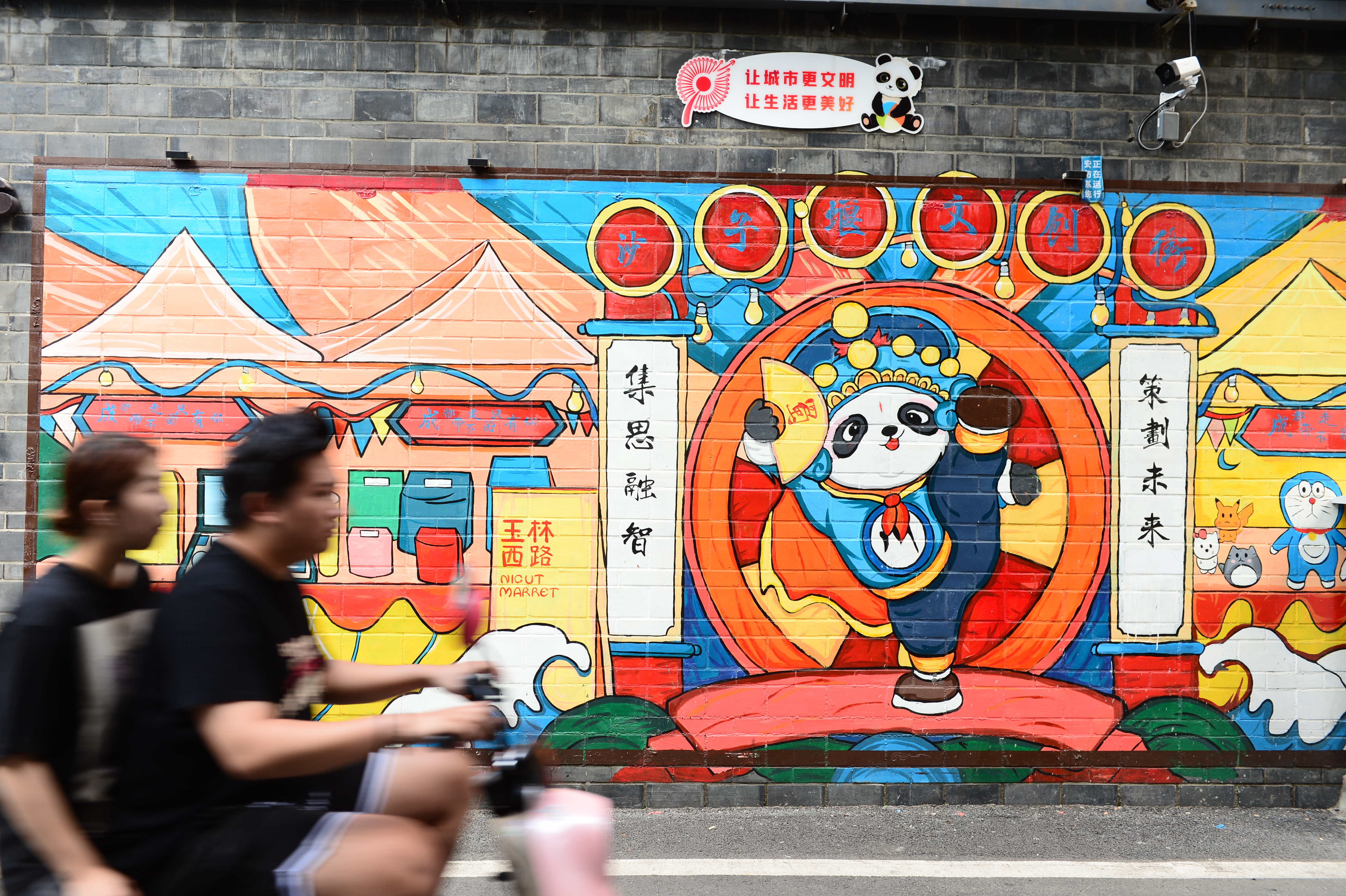This vibrant city street scene set in Asia features a brightly colored mural against a backdrop of a gray stone brick wall, which alternates between layers of wider and thinner bricks. In the foreground, a blurred image of a couple in black t-shirts is seen riding a pink scooter. The upper right corner of the wall has a white security camera positioned there, along with a white sign bearing red print in either Japanese or Chinese characters.

Dominating the mural is a dynamic scene centered around a kung-fu panda with a distinct white face, black eyes, and a red mouth. The panda, performing an agile dance move with one leg raised, is adorned in a blue sweatshirt, blue pants, brown sneakers, and a gold and blue hat with yellow round adornments. It holds a yellow fan in its right paw. Surrounding the panda is an archway composed of circular elements with red centers featuring Chinese characters, as well as two vertical banners with oriental writing.

Complementing the central figure, the mural also depicts bright circus-themed scenes. On the left, there's a shop front with the sign "NIOUT market" selling various bags. To the right, cheerful, stuffed animal caricatures, including Pikachu, Hello Kitty, and possibly Doraemon, add a whimsical touch. Above and around these elements, an orange and blue circus tent background enhances the festive feel of this bustling urban artwork.